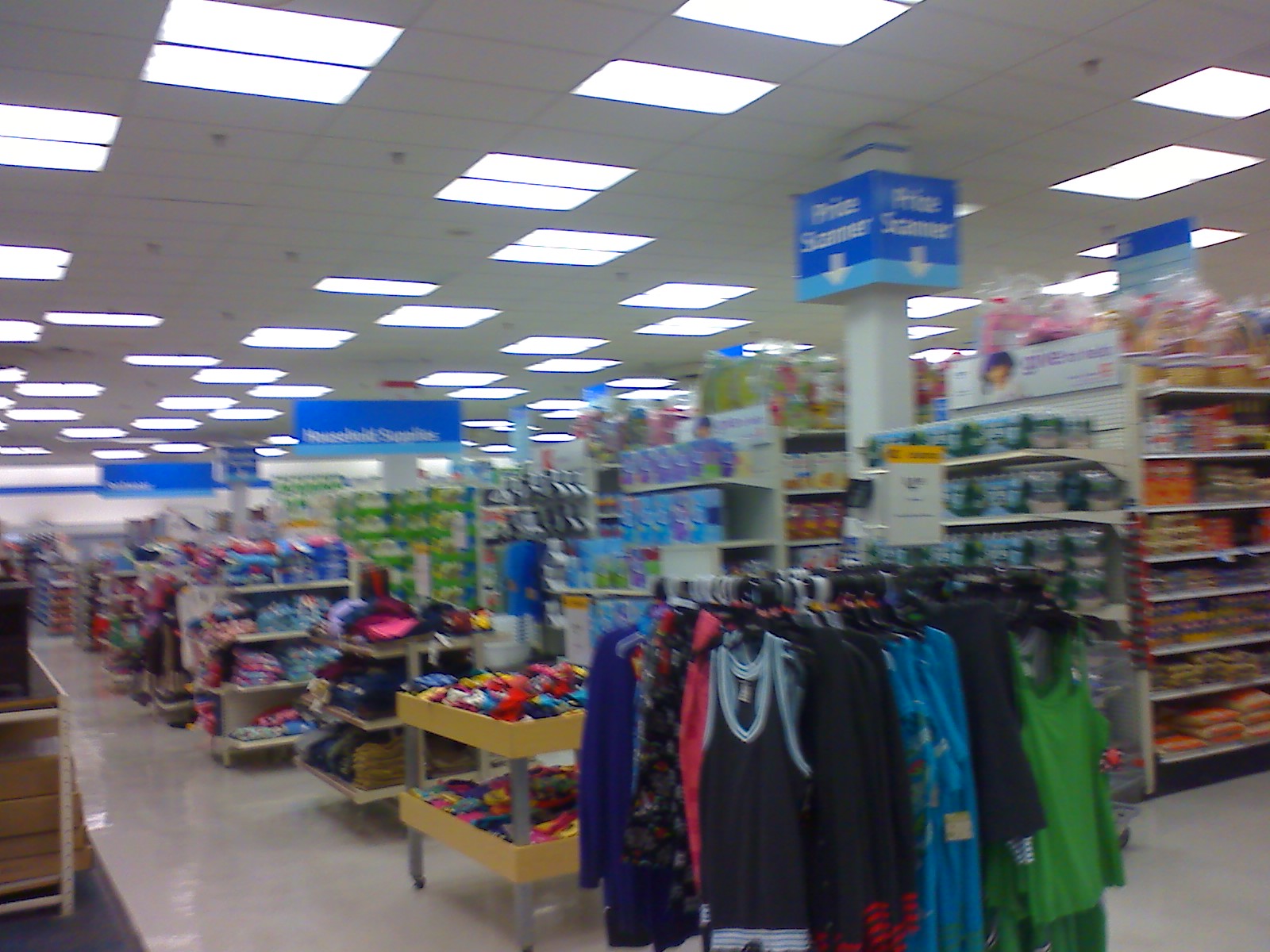The image depicts a spacious shopping center, closely resembling a Walmart or a Target. The scene captures a broad, open aisle flanked by racks of neatly arranged dresses and shirts. Adjacent to these garments is a bed dedicated to socks. Rows of aisles extend into the background, filled with an assortment of items. A sign mounted on a pole reads "Print Scanner," guiding shoppers within the store.

Shelves along the aisles are stocked with various products, and in one section, boxes of what might be toilet paper are visible. Another aisle appears to display bags of rice, indicating a diversified merchandise selection. The ceiling, adorned with bright lights, soars approximately 15 feet high, contributing to the airy and open ambiance. Numerous bins, brimming with purchasable goods, are dispersed throughout the store.

The overall atmosphere is vibrant and colorful, with hues of blue, pink, and yellow standing out prominently. The beige-tiled floors contrast with the predominantly white interior, enhancing the feeling of cleanliness and spaciousness typical of large retail stores like Walmart or Target.